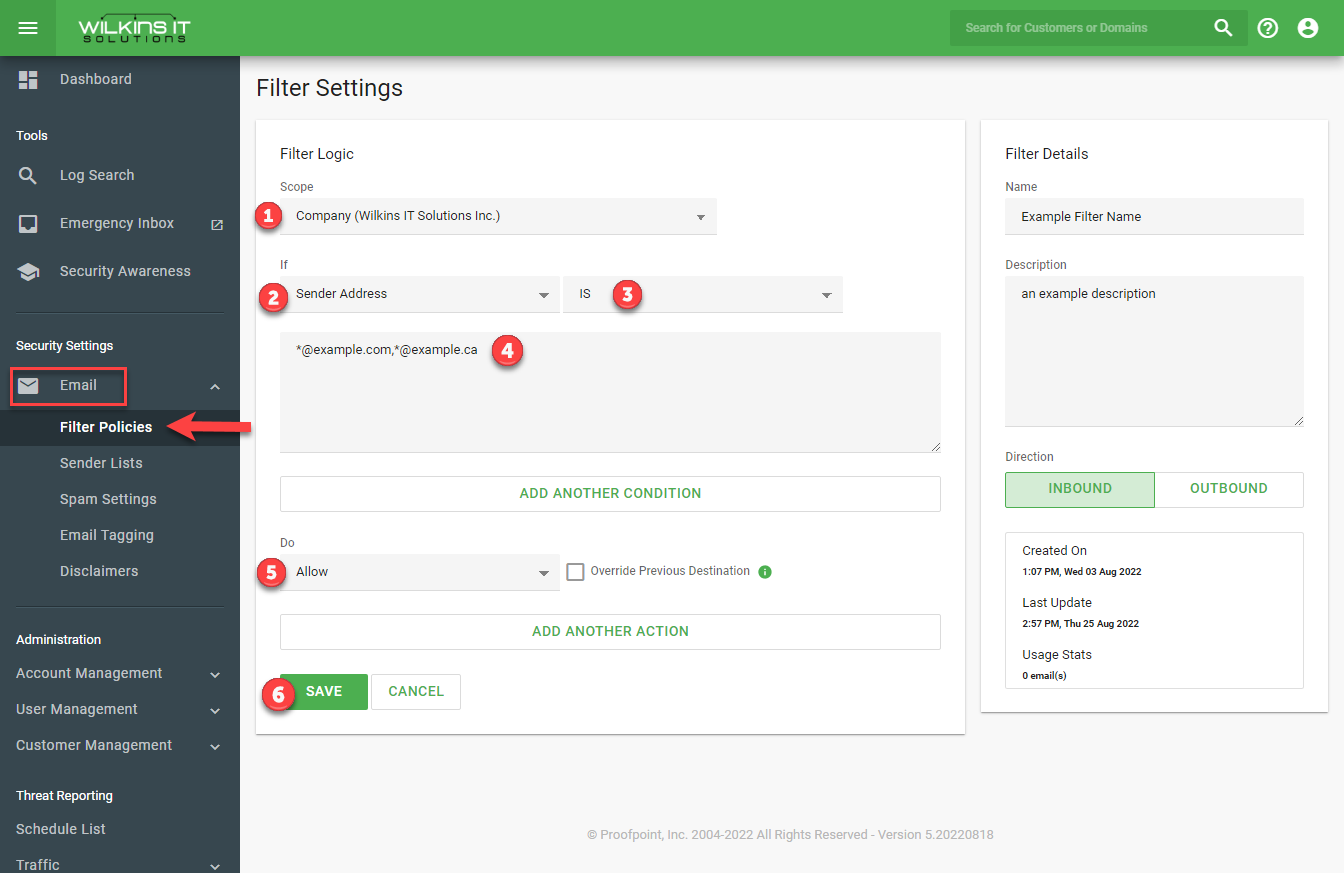**Website Interface of Wilkins IT Solutions: Detailed Description**

The screenshot captures the interface of the Wilkins IT Solutions website. At the top of the page, prominently featured, is the title "Wilkins IT Solutions." In the top-right corner, there are options labeled "Search for Customers or Domains," alongside icons for help and user profile access.

On the left side, a vertical navigation menu is visible, listing the following options: 
- Dashboard 
- Tools 
- Log Search 
- Emergency Inbox 
- Security Awareness 
- Security Settings 
- Email (highlighted with a red outline and an arrow pointing to it, emphasizing its importance)
- Filter Policies 
- Sender Lists
- Spam Settings 
- Email Tagging 
- Disclaimers 
- Administration 
- Account Management
- User Management 
- Customer Management 
- Threat Reporting 
- Schedule List 
- Traffic

To the right of this menu, several filter settings sections are delineated:
1. **Filter Settings, Filter Logic, Scope**: This area is used for defining the filter settings for email management.
2. **Company**: "Wilkins IT Solutions, Inc."
3. **Condition Builder**: Sequentially numbered steps guide the user through setting up conditions, for example:
   - **If** the **Sender Address** is **at example.com** or **at example.ca**.
4. **Actions**: The user can choose to **Allow** certain emails and **Override Previous Destination** (which is not currently selected). Additional conditions and actions can be added.
5. **Save** and **Cancel** buttons are available to finalize or discard the configurations.

To the far right, a vertical segment labeled "Filter Details" provides specific information about the filter:
- **Name**: Example Filter Name
- **Description**: Example Description
- **Direction**: Options include Inbound and Outbound
- **Created on**: 1:07 PM, Wednesday, October 3rd, 2022
- **Last Update**: 2:57 PM, Thursday, October 25th, 2022
- **Usage Stats**: 0 Emails

At the bottom, there's a footer indicating that the software is provided by **Proof Point, Incorporated**, covering the years 2004 to 2022, with all rights reserved and identifying the software version as **5.20220818**.